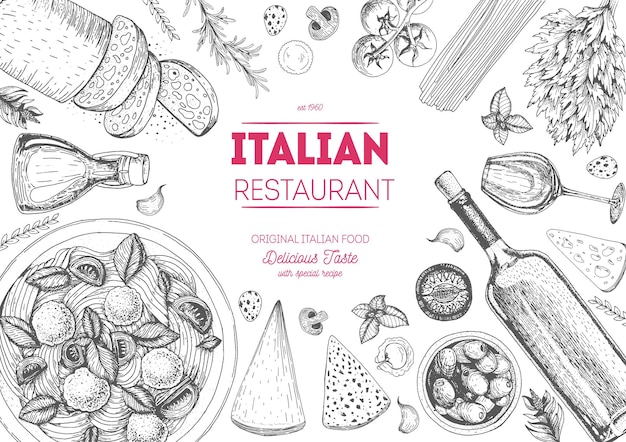The advertisement for the Italian restaurant is elegantly detailed with grayscale illustrations of various iconic Italian ingredients, creating a charming and rustic aesthetic perfect for evoking the essence of traditional Italian cuisine. The illustrations, seemingly hand-drawn in a pen or pencil style, adorn an all-white background, forming a captivating border around the vibrant center text. 

Starting at the top left corner and moving clockwise, the illustrations include sliced bread, leaves that could be basil or parsley, rosemary, quail eggs, ravioli, mushrooms, tomatoes, spaghetti, mint, a wine glass, pizza, a wine bottle with a cork, garlic cloves, olives in a bowl, various cheese like parmesan, and potentially a bowl of salad or noodles. Additional illustrations include olive oil, more leaves, and another piece of triangular bread or pizza.

In the center of the image, pink text boldly states "EST 1960," followed underneath by "Italian Restaurant" in the same color. Further down, elegant cursive text proclaims "Original Italian Food, Delicious Taste," with "Special Recipe" adding a final flourish. The juxtaposition of the monochromatic artwork with the vivid pink lettering creates a striking visual contrast that draws the viewer's attention to the restaurant's proud history and delectable offerings.